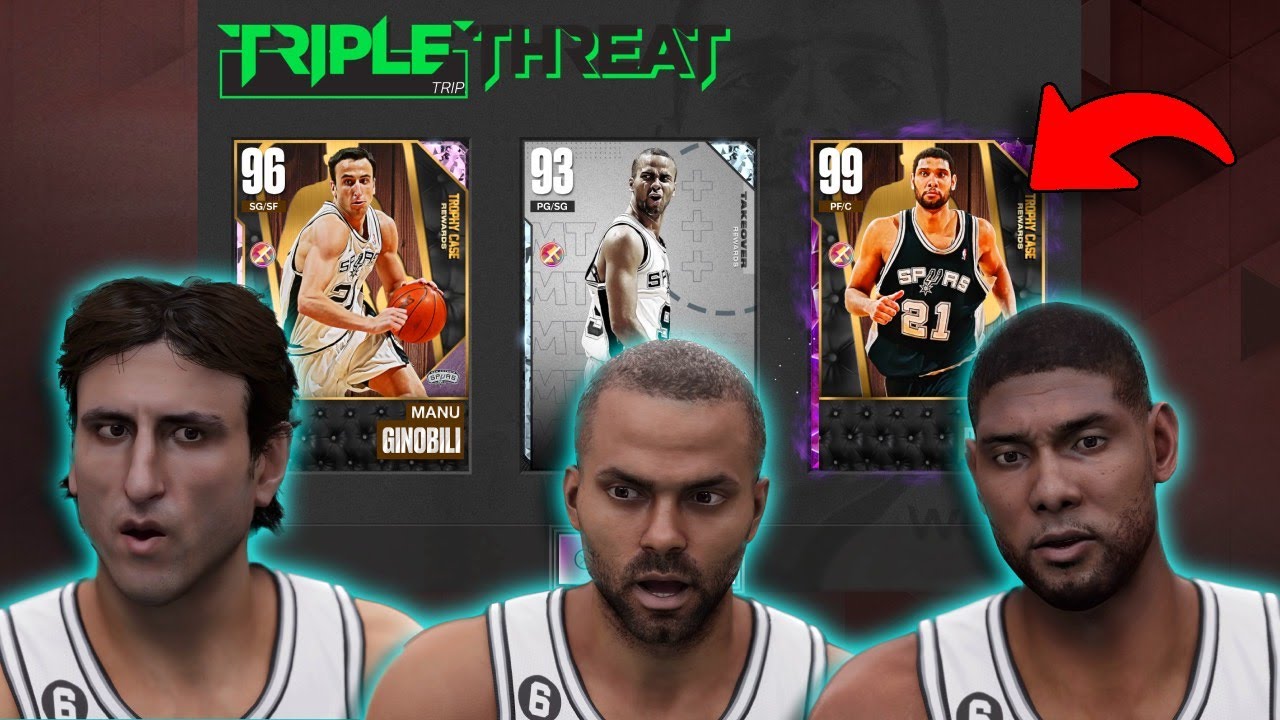In the foreground of the image, three computer-generated basketball players are prominently displayed, suggesting that this is a screenshot from a video game. Each player is depicted with detailed digital rendering, enhancing the realism yet clearly indicating their virtual nature. Behind these players are their corresponding player cards, framed in an organized layout.

At the top of the screen, vibrant green text boldly announces "Triple Threat Trip," likely the title of the video game. Each player card provides specific details: 

- The leftmost card features Manu Ginobili, wearing number 96 and holding a basketball.
- The middle card, labeled "Takeover," shows a player with number 93, though the name is obscured.
- The rightmost card displays a player wearing a Spurs jersey numbered 99, though his jersey intriguingly identifies him with number 21.

Each player in the foreground is surrounded by a turquoise halo, possibly highlighting them as selected characters or focal points. Additionally, a large, prominent red arrow points directly at the player on the right (number 99), emphasizing his significance in this scene.